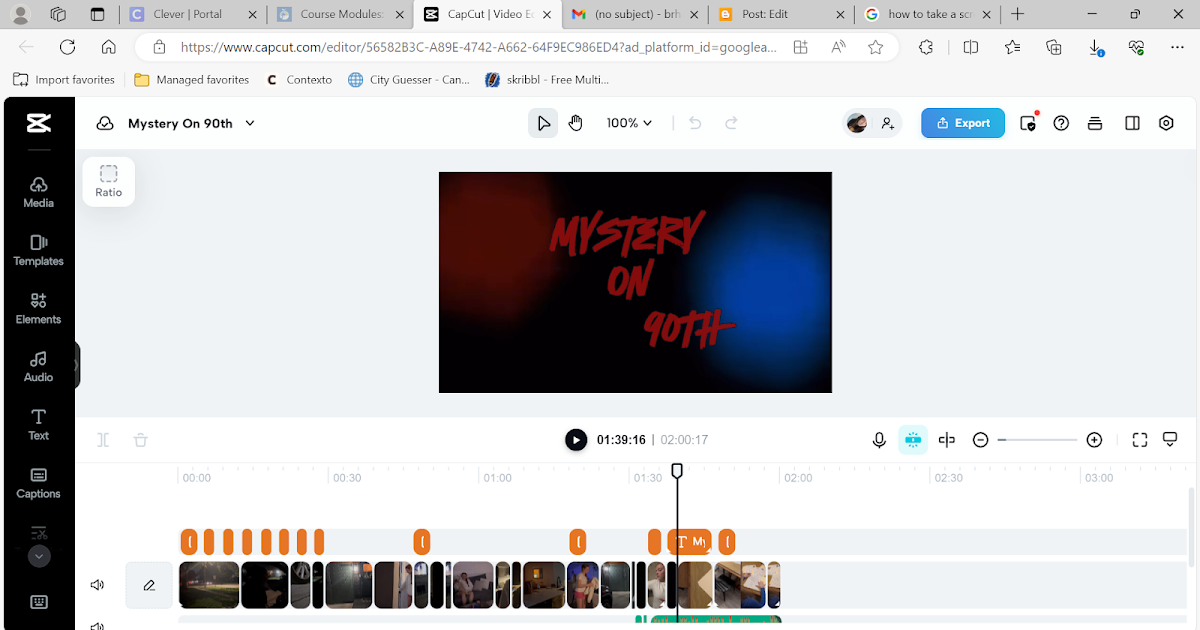Screenshot of a computer screen displaying the CapCut.com video editing webpage. The browser tab indicates the user is on the CapCut editor, with several other tabs open. The main section of the screen shows a video editing interface. At the bottom, there is a timeline with smaller thumbnail images, representing different sections of the video. The timeline cursor is positioned at the 1 minute and 39 seconds mark of a two-minute video. The current frame displayed in the preview area features the text "Mystery on 90th" on a black background. On the left side of the screen, a vertical menu presents various editing tool icons, including options for text, audio, and captions, indicating the range of functionalities available for editing.